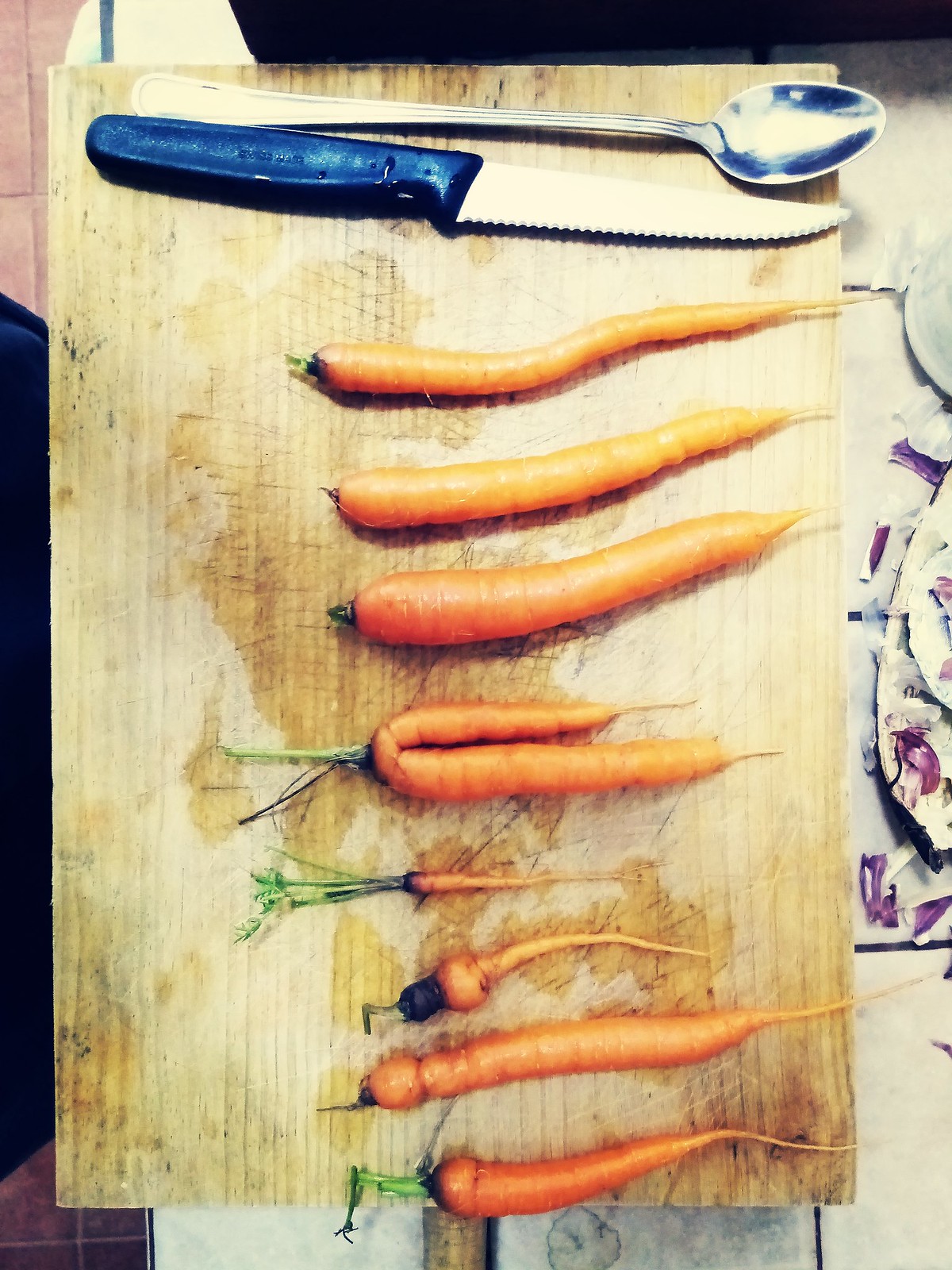The color photograph, taken indoors in portrait mode, captures a large rustic, vertical rectangular wood cutting board, clearly worn and embedded with knife marks, placed on a table adorned with a purple flower print tablecloth. At the top of the cutting board lies a silver-toned long-handled spoon, directly below which is a serrated steak knife with a black plastic handle.

Neatly lined up below these utensils are eight homegrown orange carrots, fresh from the garden, exhibiting a variety of unique shapes and sizes, indicating their uneven growth in the soil. The carrots range from tiny, pinky-sized skinny remnants to more mature, thumb-sized carrots, some extending up to eight inches long, with a mix of short green tops and darker mold at the stubs, likely to be trimmed off during preparation.

Notably, the fourth carrot from the top is distinctly unusual, forming a tight U-shape, while the two immediately below it are small and thin, resembling mini carrots. A couple of the carrots, seemingly underdeveloped, emphasize the imperfections typical of garden-grown produce. The cutting board, seemingly wet in patches, possibly from previous vegetable preparations, sets a rustic stage likely for a culinary endeavor involving these freshly picked carrots.